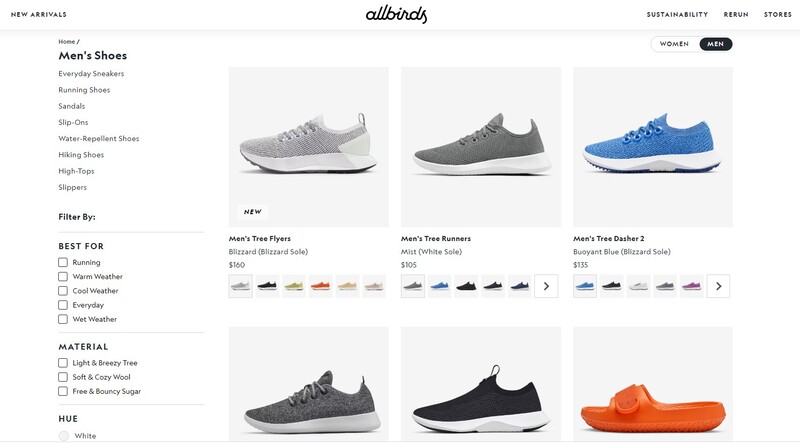The website page of Allbirds prominently features the company's logo and name at the top of the screen. On the left side, there is a navigation menu with the section titles "New Arrivals," "Men's Shoes," and a detailed clickable directory. The directory includes categories such as "Everyday Sneakers," "Running Shoes," "Sandals," "Slip-ons," "Water Repellent Shoes," "Hiking Shoes," "High Tops," and "Slippers," each provided with sub-options for filtering by "Best For," "Material," and "Hue."

On the right side of the page, adjacent to the directory, a collection of product images is displayed, showcasing various styles of men's footwear. The top row features a light gray shoe, a dark gray shoe, and a blue shoe, each characterized by a white baseline. Notably, the blue shoe's tread also incorporates a blue color. Below this row, additional products are displayed, including a charcoal gray shoe, a black shoe, and an orange slipper. The tennis shoes in this bottom row are designed with a white tread and base. Other highlighted models include the "Men's Tree Flyers," "Men's Tree Runners," and "Men's Tree Dasher 2."

Overall, the webpage focuses on a variety of sustainable shoe options, arranged for easy navigation and selection based on user preferences.